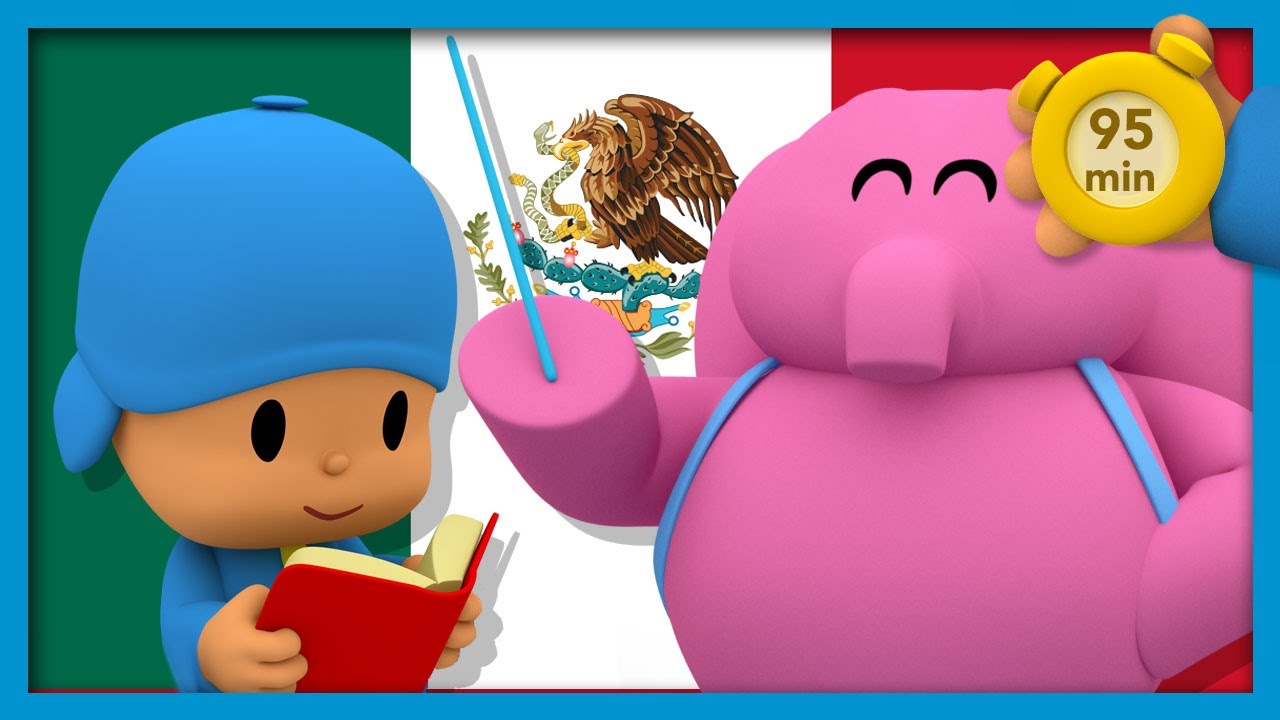In this vibrant animation, two 3D-rendered characters stand in front of the Mexican flag, which features green, white, and red vertical stripes with an eagle perched on a cactus, clutching a snake. The left character, a tan-skinned child, sports a blue cap and blue shirt while reading a red book. To the right, a large pink elephant with closed, crescent-moon-shaped eyes, suggesting a smile, holds a blue pointer stick and wears a blue backpack with front blue straps. The scene is framed by a bright blue border. In the upper right corner, a hand appears to hold a stopwatch displaying "95 minutes." This image, reminiscent of the whimsical style seen in the Pocoyo series, blends educational and playful elements seamlessly.